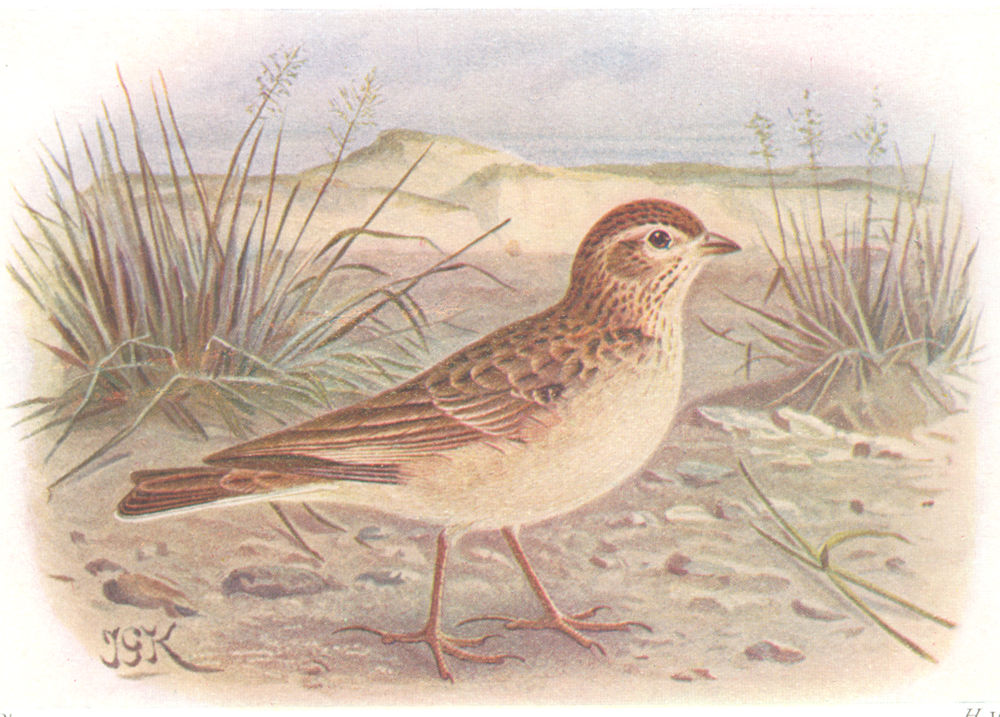This detailed image, likely an artwork—perhaps a lifelike painting, drawing, or digital creation—depicts a brown bird standing on sandy, uneven ground sprinkled with small stones. The bird, centered in the rectangle with rounded corners, features a small yellow beak, a dark brown top, and a lighter brown or white belly. It has dark brown eyes and beige or dark orange feet with three toes on each. Tall, reed-like grasses with green and brown stalks surround the bird, growing higher than it. The background reveals a vast, seemingly desert-like plain with scattered hills and dunes. The sky above is overcast with clouds, suggesting either an early morning or evening light, and there’s a hint of blue water visible behind the sandy expanse. The scene includes a white border around the edges, hinting at a possible screen capture. In the lower left corner, the initials "JGK" identify the artist. The colors used are muted, primarily featuring tans, browns, greens, blues, and grays, creating a serene yet somber natural setting.